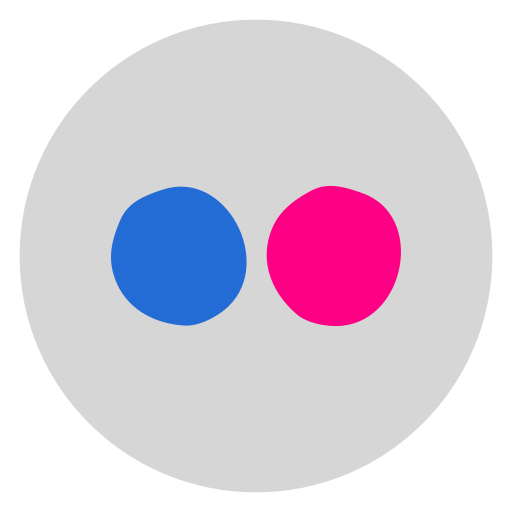The image features a minimalist design with a total of three circles set against a plain background, devoid of any text or additional imagery. The primary figure is a large, uniform, light-to-medium gray circle. This circle is perfectly rounded with smooth and regular edges, providing a solid backdrop for the inner elements. Within this large gray circle, there are two smaller, slightly irregular circles placed side by side, equidistant from the outer edge and symmetrical in their positioning.

The circle on the left is medium blue, characterized by its uniform color but slightly irregular edges. The circle on the right mirrors this irregularity but is distinctively colored in a uniform reddish-pink hue. Both inner circles are of roughly equal size and maintain the same distance from the top of the large gray circle, enhancing the balanced and symmetrical appearance. 

In summary, the visual composition is straightforward yet deliberate, presenting three distinct circles with subtle variations in edge regularity and color, set within a clean, text-free layout.